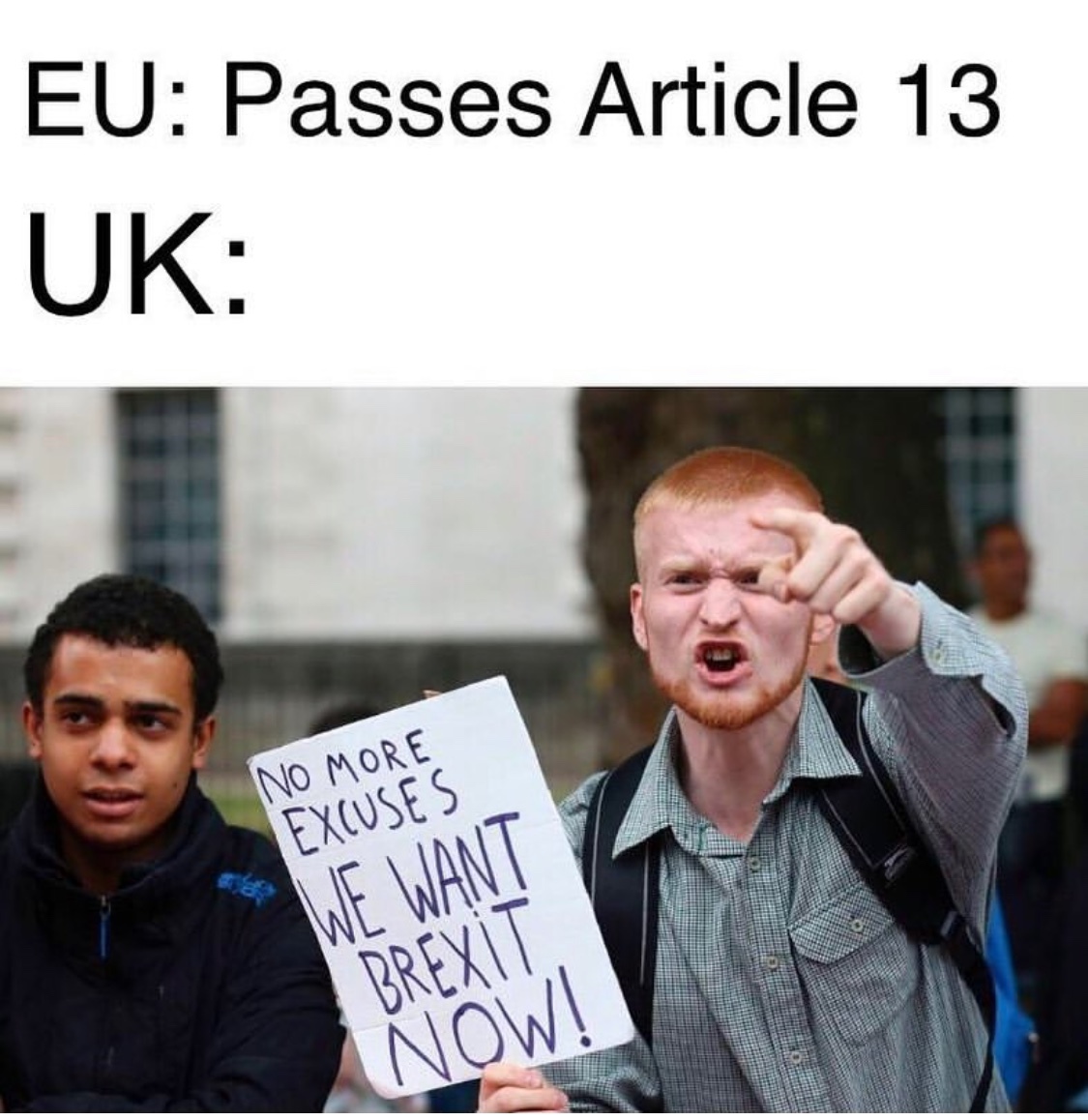The photograph is a landscape-oriented color image overlaid with black text that reads "EU passes Article 13: UK." The scene captures two young men at a protest, likely outside a government facility. The man on the right, with short red hair, a goatee, and a small mustache, has an angry expression and points his left finger toward the top left of the image. He is wearing a light blue checkered shirt with a pocket and a dark blue vest-style backpack with black straps. In his right hand, he holds a white vertical poster board with bold black text that reads, "No more excuses! We want Brexit now!" On the left, a dark-skinned man with black hair wearing a blue jacket with a light blue zipper and writing looks on towards the same direction. Behind the protestors, a building with a white stucco finish and several unfocused windows can be seen, accentuating the outdoor setting of the protest assembly. The photograph vividly captures the intensity and emotion of the moment.